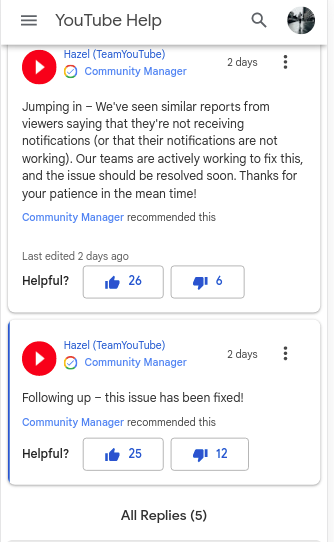**Caption:**

A screenshot of a YouTube help screen, likely taken from a mobile device, as suggested by the column layout. The screen features a user interface with several key elements:

- At the top left corner, three horizontal lines, commonly known as a 'hamburger menu,' indicating additional options.
- The header displays the text "YouTube Help," alongside a magnifying glass icon, which is typically used for searching.

Below the header, a post by "Hazel, Team YouTube Community Manager," is visible, dated two days ago. The content of the post addresses an issue users have reported about not receiving notifications:

> "Jumping in, we've seen similar reports from viewers saying that they're not receiving notifications or that their notifications are not working. Our teams are actively working to fix this, and the issue should be resolved soon. Thank you for your patience in the meantime. Community Manager recommended this."

This post was edited, indicated by "Edited last edit two days ago." Interactions with this post show it has 26 helpful votes and 6 not helpful votes. 

Another entry by Hazel follows this:

> "Follow-up: This issue has been fixed. Community Manager recommends this."

This update has garnered 25 helpful votes and 12 not helpful votes. Additionally, there are 5 replies to this update.

The major colors on the page include a white background with black and blue text, where blue likely represents hyperlinks. Interaction buttons, such as thumbs up and thumbs down, are accompanied by numbers in blue. The red circles with white arrows pointing to the right likely signify navigation or action buttons.